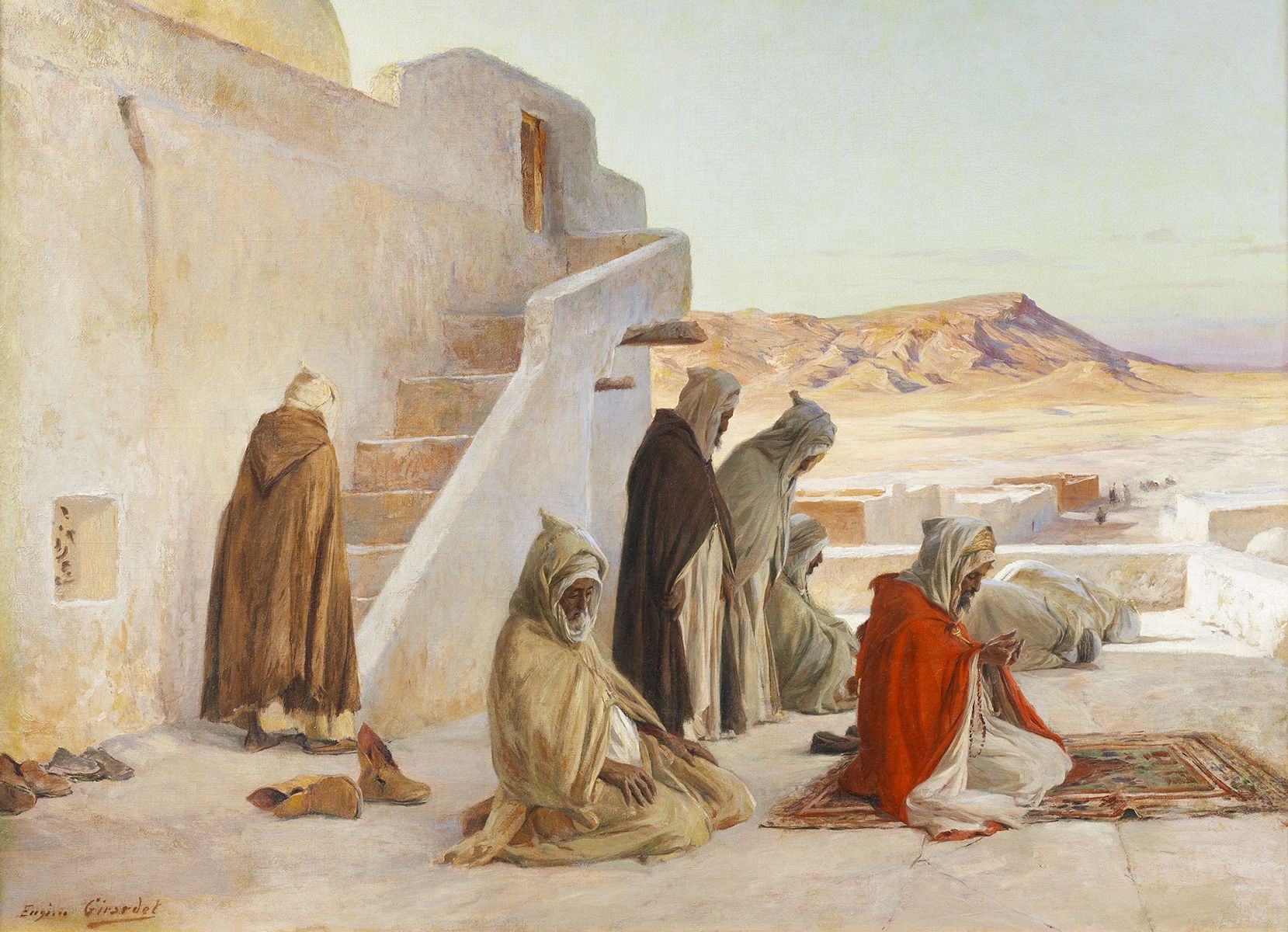The image is a detailed painting set in a desert landscape under a clear blue sky, featuring a group of at least six to eight men in various states of prayer. These men are gathered in front of an adobe-style house, characterized by its cement-like structure with protruding wooden beams and stairs leading to an upper level. The building sits within a desolate area marked by rocky formations or dunes, devoid of any plant life. 

All the men are dressed in long, flowing robes primarily in shades of white, cream, brown, red, and black, with some wearing hoods. They have removed their shoes, which are piled at the base of the stairs. Several men are kneeling on ornately decorated prayer rugs, deeply engrossed in their prayers, with heads bowed or fully kneeling. A lone figure can be seen ascending the stairs at the back. The color palette of the painting consists mainly of earthy browns and whites, with the vibrant hues of their robes adding contrast. The scene exudes a serene, contemplative atmosphere as the men stand, kneel, and bow in reverence against the backdrop of their stark, desert environment.